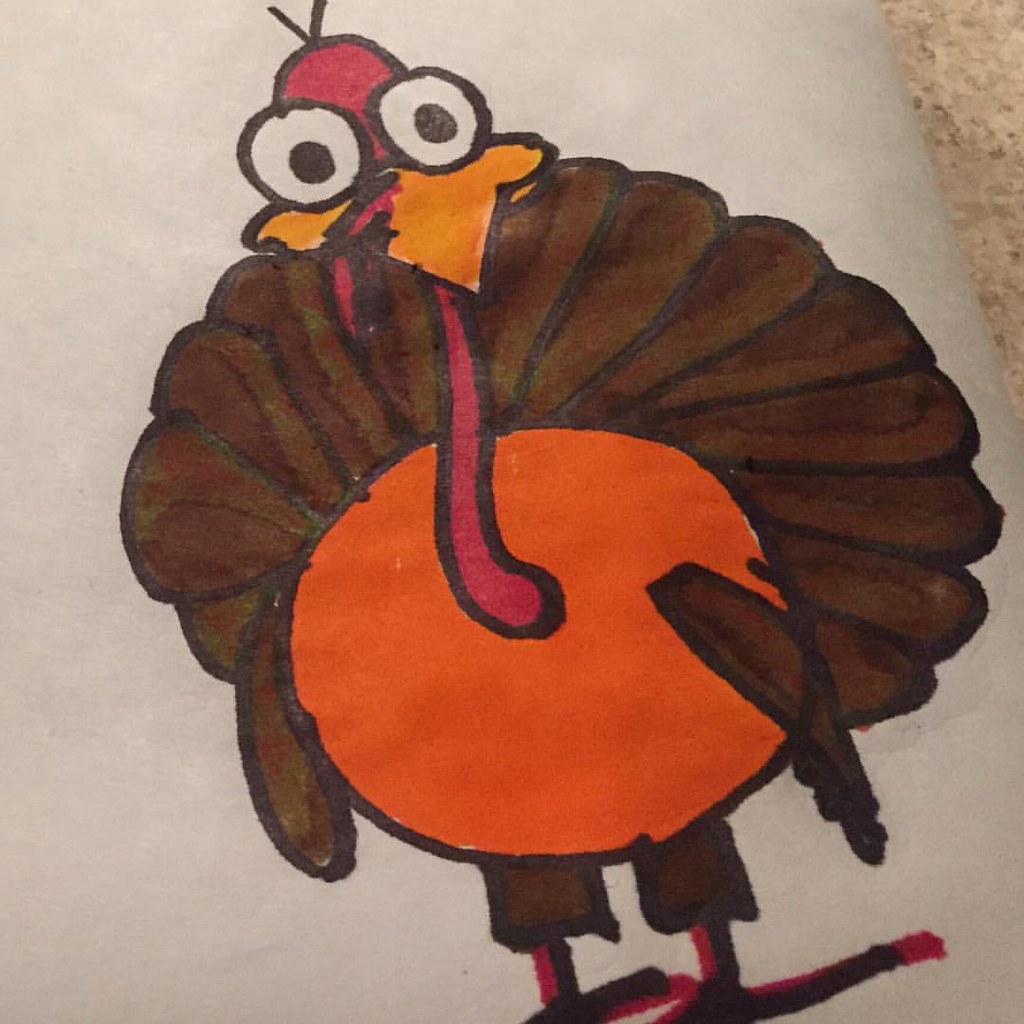This artwork features a vibrant and whimsical drawing of a turkey, rendered in thick black marker. The turkey's body is prominently colored in orange, while its feathers are showcased in rich brown hues. The bird is adorned with a large, fan-like tail and simplistic stick-like legs, which are depicted as black lines with a red outline. This playful illustration highlights a yellow beak and oversized, cartoonish eyes, adding a touch of character to the turkey. The head is distinctly red. Notably, there appears to be a small artist's error near the beak, where an unintended red section is visible, resembling an additional piece of the neck. This minor discrepancy adds to the charm and unique nature of the drawing.